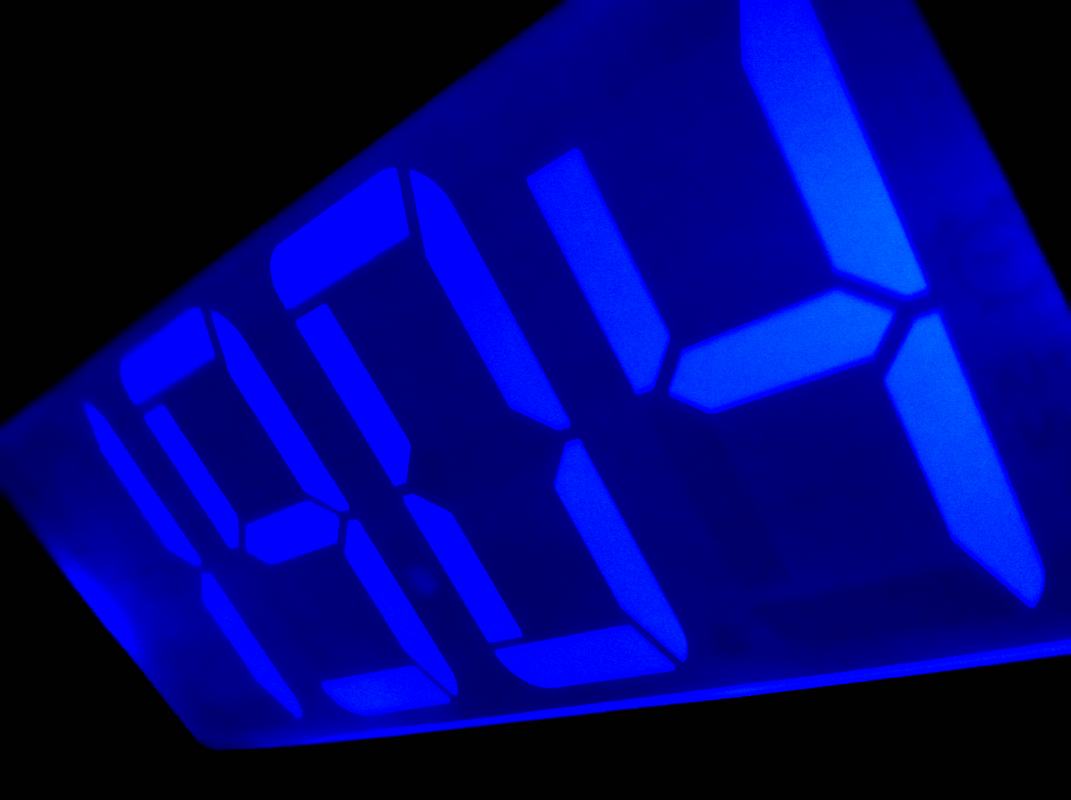A striking photograph captures an immense digital clock display set against a pitch-black backdrop. The display, illuminated in a dark blue hue with white numerals, prominently shows the time as 19:04, indicating 7:04 PM in military time. The stark contrast between the glowing blue digits and the dark background enhances the clarity and prominence of the time. The minimalist composition focuses solely on the clock, devoid of any additional decorative elements, emphasizing the interplay between the luminous display and the surrounding darkness.